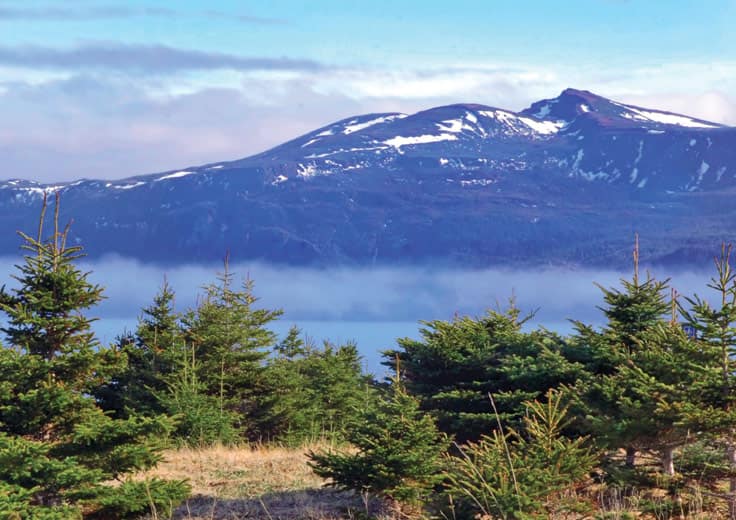The photograph captures a stunning mountain range with snow scattered across the upper peaks, set against a backdrop of a light powder blue sky with patchy white and gray clouds. The mountains stretch across the entire width of the image, with fog or mist lingering at the base, indicating a high altitude. At the very bottom of the photo, green and brown grassy areas frame the scene, interspersed with small evergreen trees that resemble Christmas trees, standing about five feet tall. The foreground features a mix of green bushes and some dried-out grass, adding layers to the natural landscape. No identifiable landmarks, animals, or people are present in the image, and a small marking can be noted in the bottom left corner of the photograph.